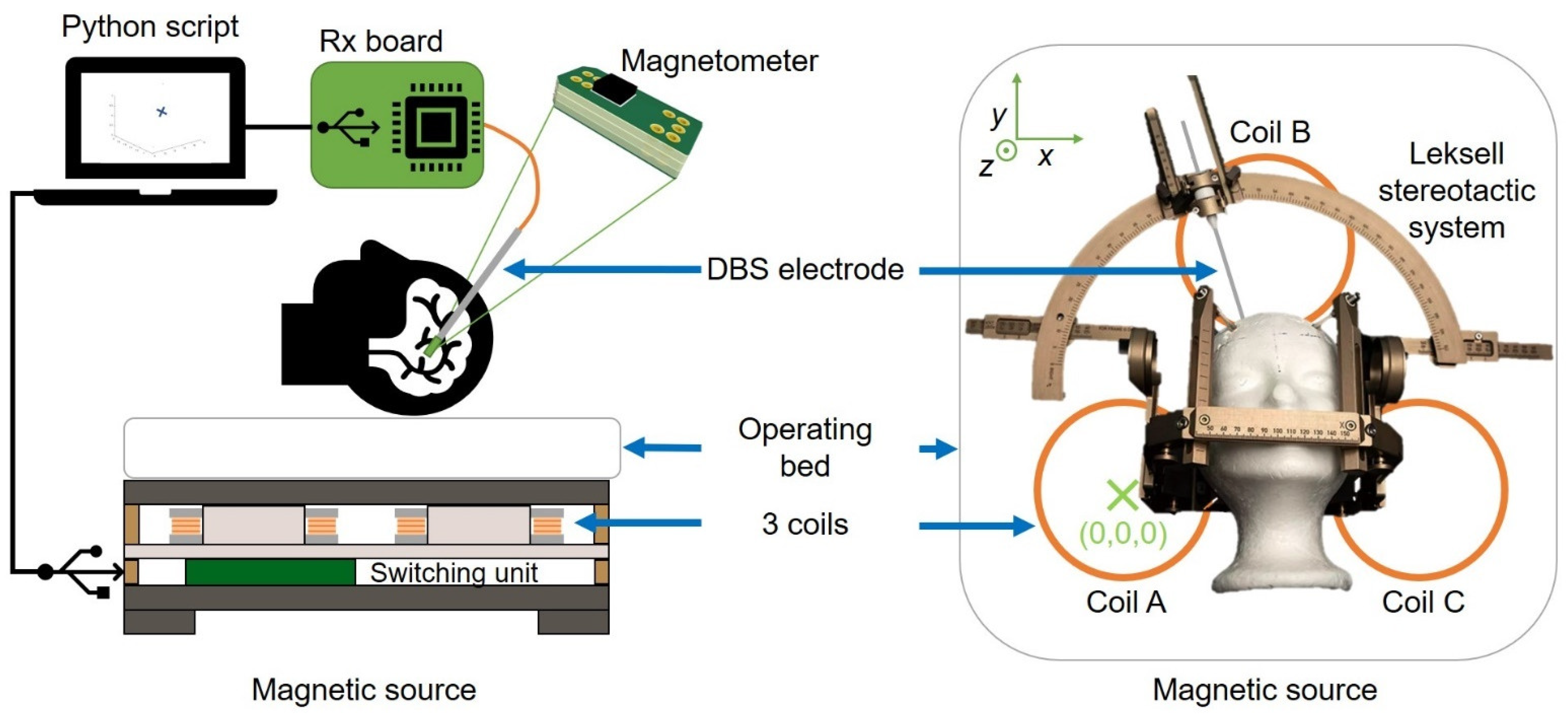This diagram depicts a detailed process likely related to a study on the human brain, centered around the use of magnetic sources and DBS (Deep Brain Stimulation) electrodes. 

In the top left corner, there is a laptop labeled "Python Script," which connects via a line to a green box labeled "RX4." Beneath this, a pink line extends downwards to a white-brained silhouette of a human head. 

Above the head, there's a label "Magnetometer." Below the head, an electronic box labeled "Switching Unit" is connected to another label "Magnetic Source." Extending to the right of the head, lines point towards labels "DBS Electrode" and "Operating Bed" with blue arrows moving in both left and right directions.

Further down, "3 Coils" are indicated with additional electronic components on the diagram. Towards the right side, there's a white dummy head labeled with details "Coil B" and marked under the "Vexcel Stereotactic System." To the left, "Coil A" is enclosed within an X and outlined circle, and on the right, another circle labeled "Coil C." Both magnetic sources flank the diagram titles "Magnetic Source," connected with the unified process of DBS electrodes and studying brain activity.